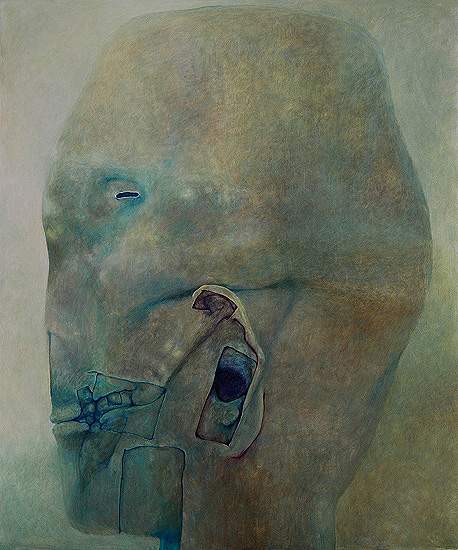The artwork presents a modernist, abstract painting of a humanoid face that closely resembles a carved stone head. The head is facing left and is depicted primarily in neutral, muted colors such as drab gray, olive, and greenish-brown, with occasional hints of yellow, blue, and off-white. The face has an elongated, oval shape with multiple irregularities and distortions. Notably, the eye is represented by a narrow slit within an empty socket, and part of the flesh around the mouth is absent, exposing the teeth. The jawline and ear region also appear fragmented and damaged, adding to the impression of a weathered, monumental stone sculpture. The background echoes the painting's earthy tones, blending shades of green and brown to reinforce the somber and subdued atmosphere of the piece.